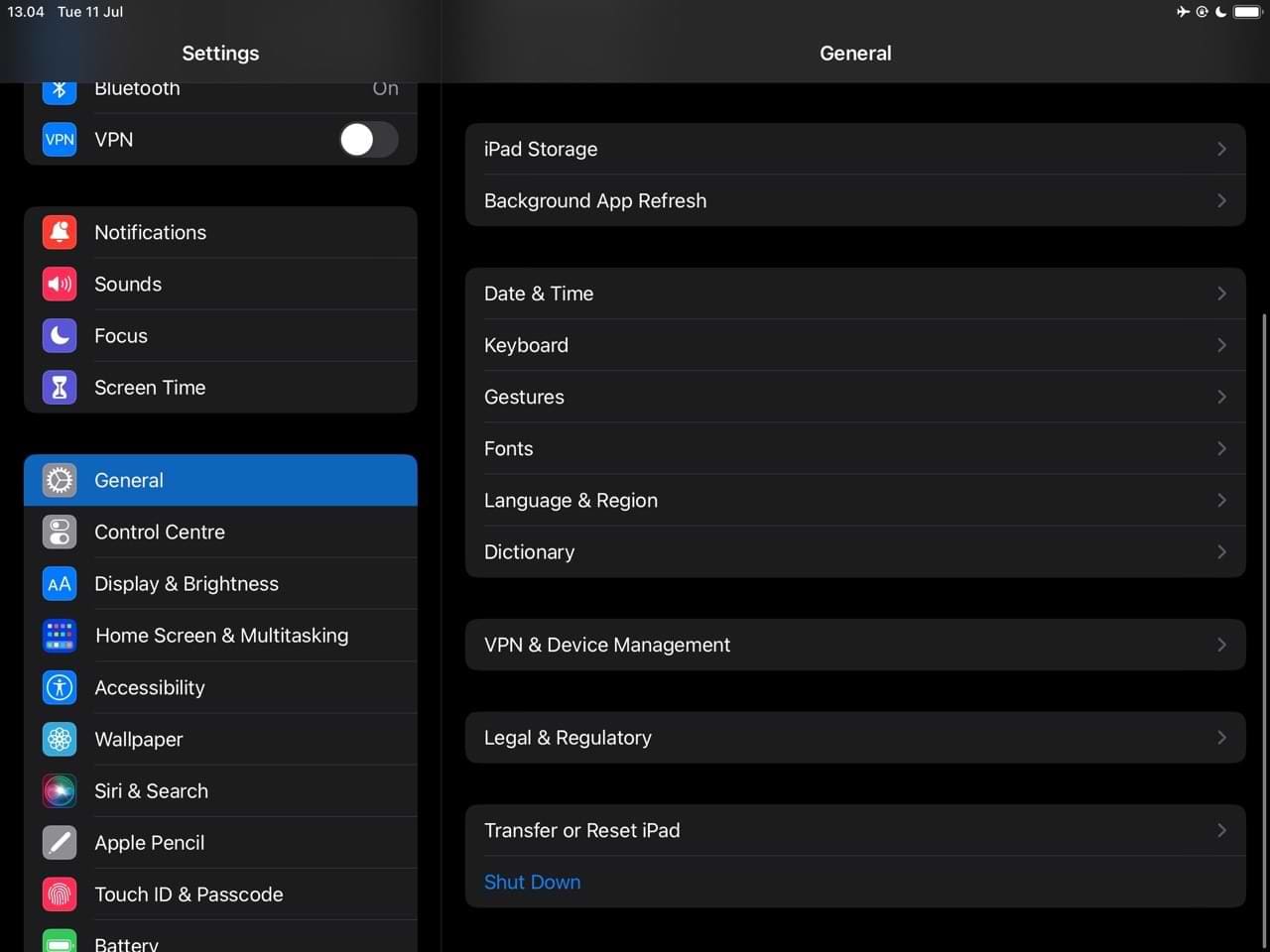The image displays the settings menu of an iPad, showcased in landscape mode with a wider layout, suggesting it is indeed a tablet rather than a phone. The device is set to dark mode, featuring a black background and white text. Key options visible in the menu include Bluetooth, VPN, Notifications, Sounds, Focus, Screen Time, General, Control Center, Display & Brightness, Home Screen, Accessibility, Wallpaper, Siri, Apple Pencil, Touch ID, and Battery. Notably, the presence of the Apple Pencil option further indicates it's an iPad. The general settings have been clicked, revealing additional options on the right side such as iPad Storage, Background App Refresh, Date & Time, Keyboard, Gestures, Fonts, Language, Dictionary, VPN, Legal, Transfer or Reset iPad, and Shutdown.